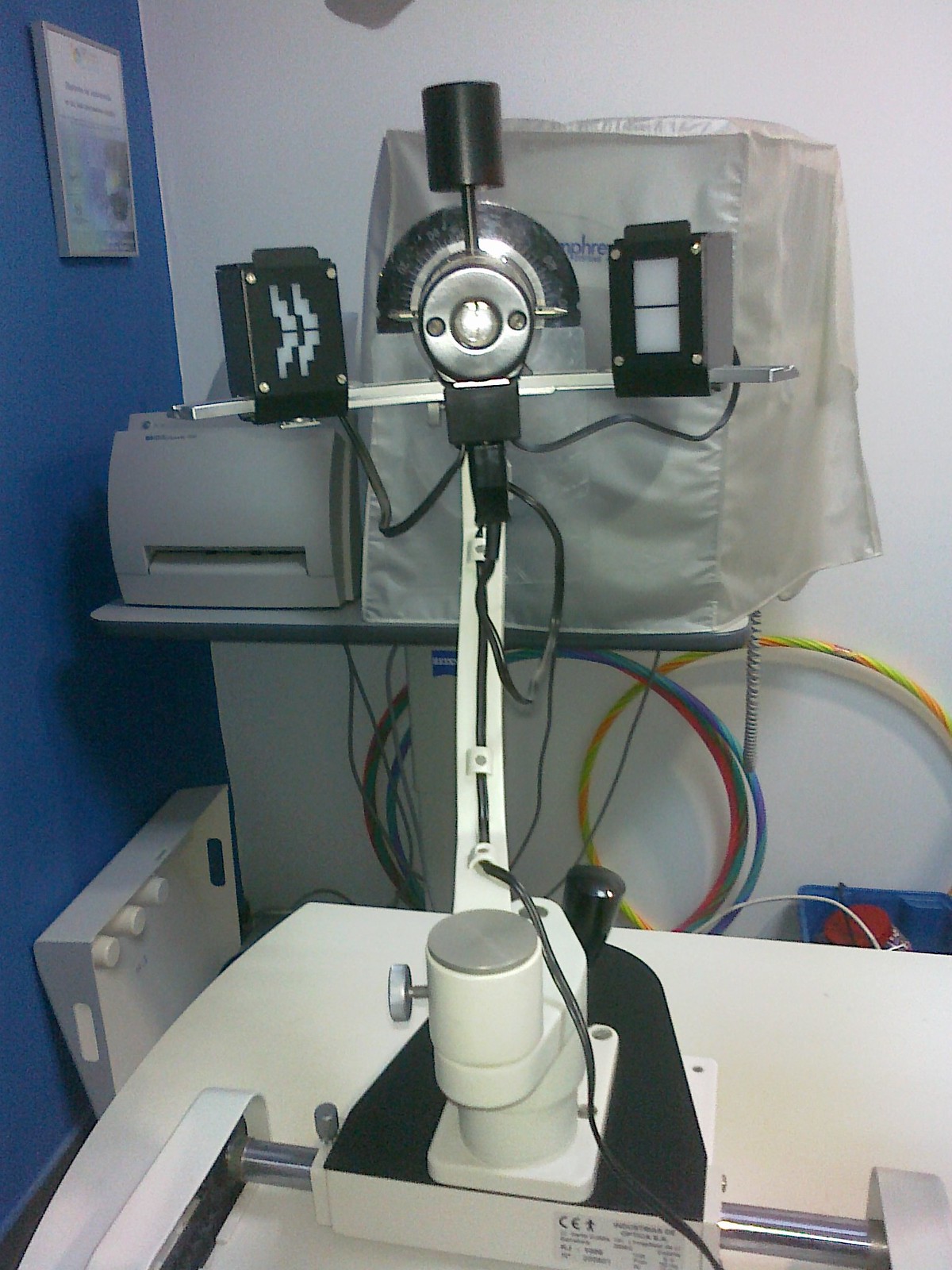The image depicts a sophisticated, professional-looking medical device situated on a white table, positioned in the corner of a room. The device features a long stem with various components extending upwards, resembling a cross. It includes two black boxes with white elements in the middle on one side, and some type of graphic or screen on the left side. At the pinnacle of the device, there is a prominent silver meter, potentially adjustable, with additional elements projecting from the top. Dangling from the device are three colored cables—blue, red, and yellow—likely used for connecting to other equipment.

In the room's background, miscellaneous items can be seen: three colorful hula hoops leaning against a wall, a white printer, and another covered machine suggesting specialized usage. Additionally, a lid that appears to belong to the medical device is positioned by the wall, while a poster or picture is visible in the upper left corner. The setting conveys a clinical yet cluttered atmosphere, indicative of a multi-functional workspace.